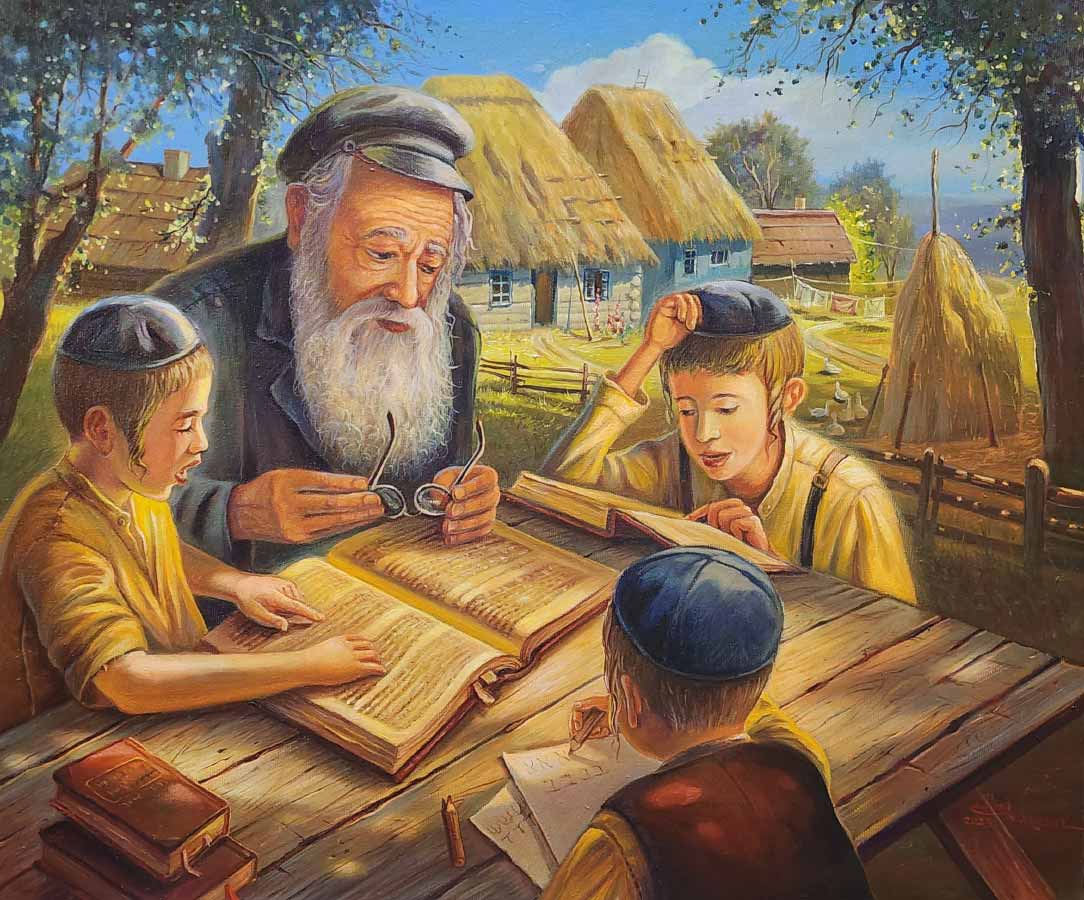In the foreground of an old-time village with log and stone houses featuring thatched roofs, a wooden table is surrounded by a scene of Jewish tradition and learning. The table is set at an angle, with the old man, who has a long white beard and grayish eyebrows, seated at the top left corner. He wears a black cap and a black jacket, and holds his glasses between his hands. Around him are three young Jewish boys, identifiable by their yarmulkes. The boy on his left, dressed in a yellow polo shirt and long hairlocks hanging down, points at a section of an open, thick book they are studying together. Another boy across from the old man is actively writing something in Hebrew on a white piece of paper. To the old man's right, another child, also in a yellow shirt but with suspenders, is engrossed in reading his own book. A stack of biblical books can be seen in the lower left corner of the scene. The background showcases the simple life of the village, with homes featuring grass and straw roofs, a barn, a clothesline, and a haystack, completing this snapshot of intergenerational learning and cultural heritage.